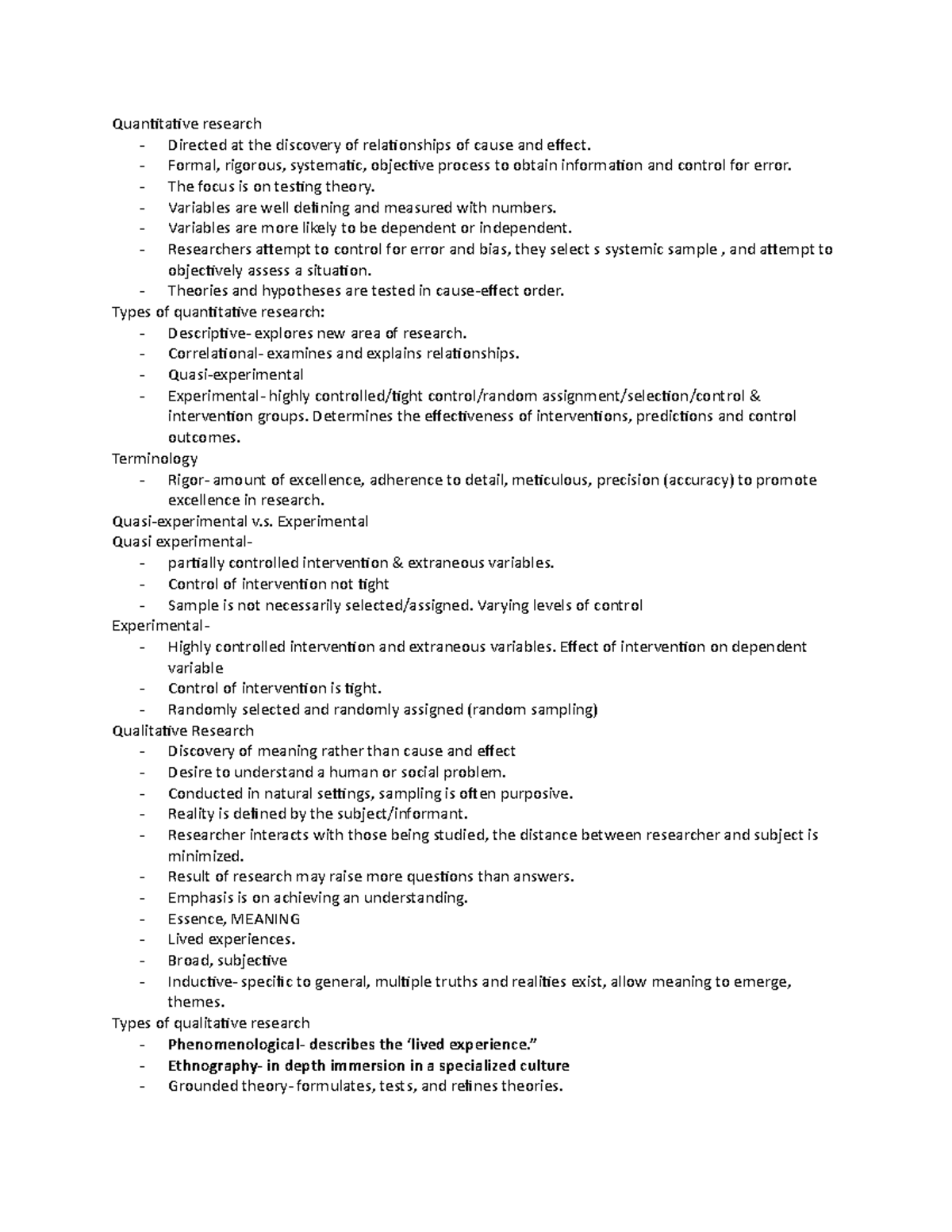The image features a white background adorned with a collection of black text. The text is quite small and somewhat blurry, making it challenging to read. The content of the text appears to focus on the domain of quantitative research, outlined through a series of concise points. Here is a detailed breakdown of the text:

1. **Quantitative Research:**
   - Directed at the discovery of relationships of cause and effect
   - Formal, rigorous, systematic, and objective process to obtain information and control for error
   - The focus is on testing theory
   - Variables are well-defined and measured with numbers
   - Variables are more likely to be dependent or independent
   - Researchers attempt to control for error and bias
   - Researchers select a systematic sample and attempt to objectively assess a situation
   - Theories and hypotheses are tested in a cause-effect order

2. **Types of Quantitative Research:**
   - Descriptive: Explores new areas of research
   - Correlational: Examines and explains relationships
   - Quasi-experimental: Involves some manipulation of variables but lacks random assignment
   - Experimental: Involves manipulation of variables and random assignment to control for variables

This refined caption offers a comprehensive overview of the key aspects and various types of quantitative research, emphasizing its structured and methodical nature aimed at establishing cause-and-effect relationships and testing theories.